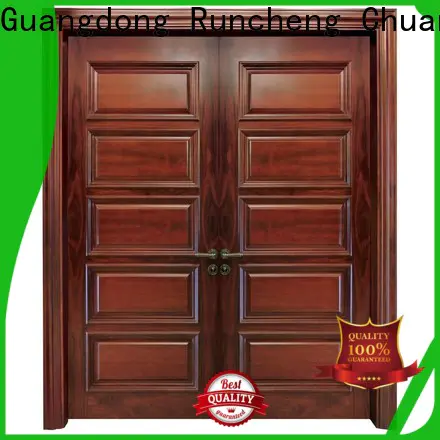This image is a computer-generated advertisement showcasing a set of elegant wooden double doors, framed against a pristine white background with a vivid green border. The doors, crafted from rich, dark brown wood with a polished finish, feature five vertical rectangular panels on each side. Central to their design are intricate brass or bronze latch handles located near the middle, complemented by circular locks beneath. The top of the image bears the black text "Guangdong Runcheng Chua," likely indicating the brand or manufacturer. At the bottom, there are two prominent labels: the center one is a circular, red, and white badge that reads "Best Quality," resembling the top of a ribbon, while the right side displays a red shield with a gold outline, stating "Quality 100%," underscored by a red ribbon at the bottom. The overall presentation emphasizes the high quality and craftsmanship of the doors.